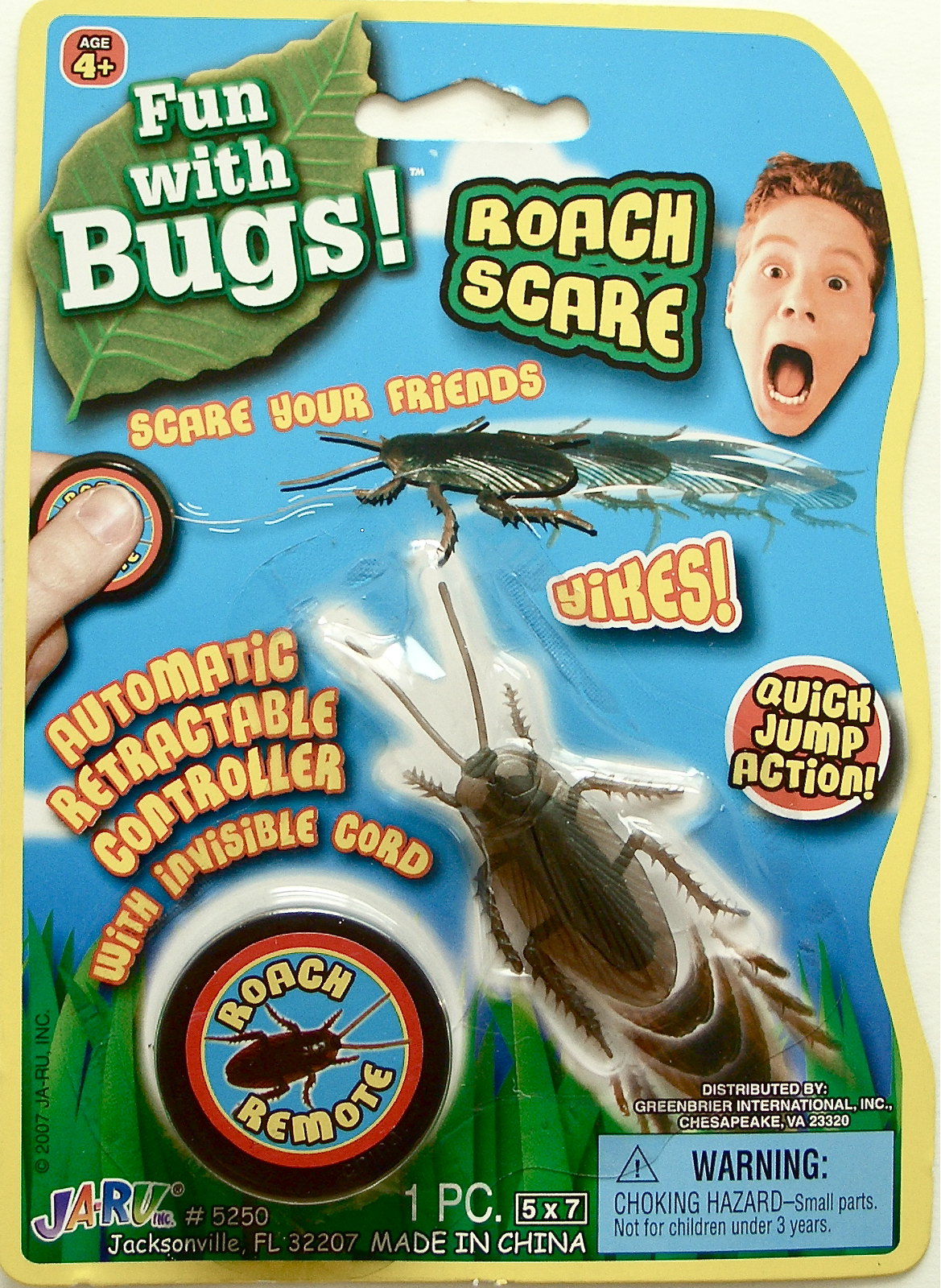This vertical, scallop-edged image appears to be the cover of a vibrant toy packaging, possibly a magazine cover, positioned for a toy targeted at children. Dominated by bright, eye-catching colors such as yellow, green, red, orange, light blue, purple, and brown, the package effectively grabs attention. 

In the upper left corner, a leaf-shaped design in big white letters reads "Fun with Bugs!" To its right, an alert in yellow letters on a green background states "Roach Scare!" Next to this is an image of a boy with auburn red hair, his mouth open in a scream, reacting to the bugs. Below in slightly smaller yellow letters is the phrase "Scare Your Friends!" Further down is a large image of a bug, and beneath this, in bold yellow letters with a red border, the word "Yikes!" These phrases are surrounded by dynamic descriptions such as "Quick Jump Action," "Automatic Retractable Controller with Invisible Cord," and "Roach Remote."

A visibly large hand enters from the left side of the image, perhaps demonstrating the toy's interactive nature. On the bottom right, another significant bug image is strategically placed. The blue background at the top transitions into a grassy bottom, adding a playful outdoor touch. Additional text includes "distributed by Greenbuyer International" and a small tagline at the bottom that reads "JARV, Jacksonville, Florida, made in China. One piece, five by seven." The whole design vividly presents an exciting toy concept designed to thrill and entertain children ages 4 and up.